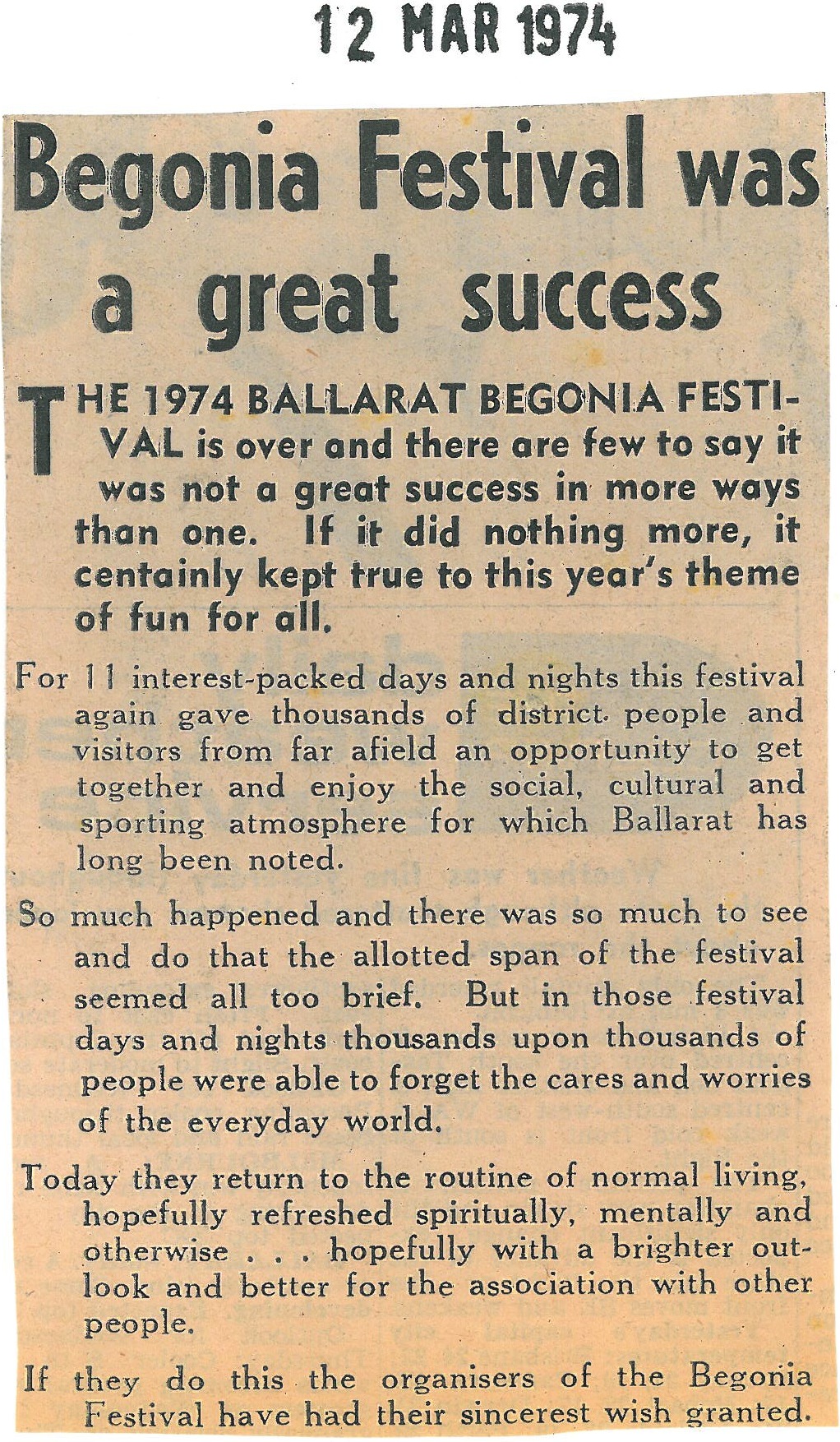This image depicts a newspaper clipping dated 12 March 1974, featuring an article titled in bold text "Begonia Festival was a great success." The faded off-white or beige-tan paper, along with the old-style black font, gives it a distinctly dated appearance. The article celebrates the 1974 Ballarat Begonia Festival, highlighting it as an overwhelming success that stayed true to its theme of "fun for all." For 11 days and nights, the festival provided thousands of local residents and visitors from distant places with abundant opportunities to engage in social, cultural, and sporting activities, showcasing the unique atmosphere Ballarat is known for. Despite the brief span of the festival, it allowed countless attendees to momentarily escape their daily worries and routines, returning to their lives spiritually and mentally rejuvenated. The organizers' most heartfelt wish appears to have been fulfilled, leaving participants with a brighter outlook and enhanced communal connections.